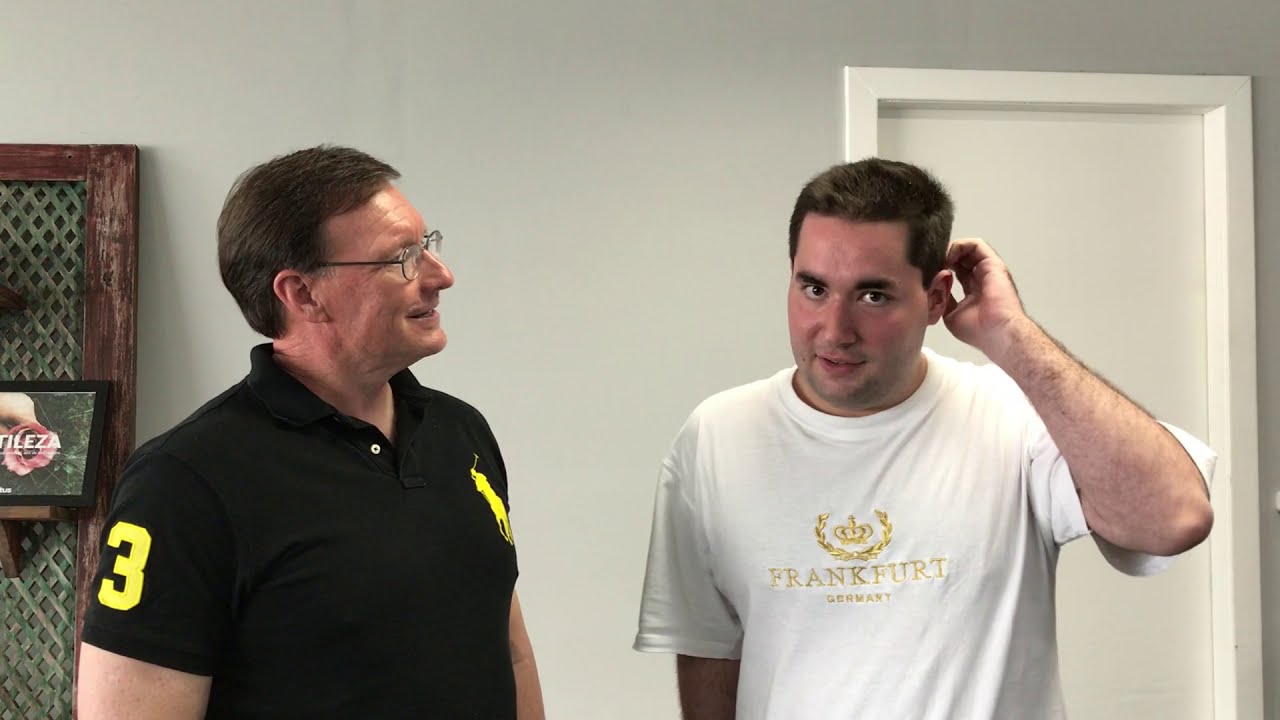In a cozy living room, a detailed photographic image captures two Caucasian men, clearly of different generations. The older man, positioned on the left, appears to be in his 40s and has brown hair. He is wearing glasses and a black polo shirt with a distinctive yellow logo and the number 3 on his right sleeve. He gazes with a smile at the younger man standing to his right. The younger man, who has brown hair and a slightly chubby face, is dressed in a white t-shirt emblazoned with the words "Frankfurt, Germany" in gold, along with a crown logo. This man, positioned in front of a closed white door in a grey-walled room, has his left hand raised towards the back of his head and is looking directly at the camera. To the older man's left, partially seen, is a bookcase or shelf unit that holds a decorative sign with the acronym "N-L-E-Z-A," featuring a brown frame and a green center depicting a flower and a hand. The setting exudes a personal and relaxed atmosphere.